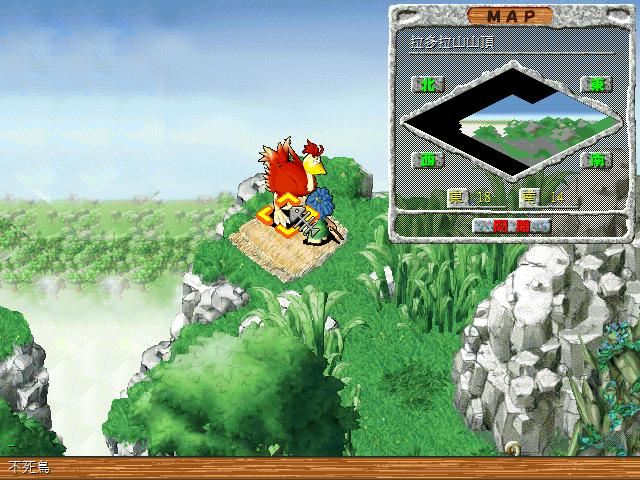The image appears to be a scene from an old video game reminiscent of the style seen on the Super Nintendo console. At the top of the image, a blue sky with hints of white suggestive of clouds stretches across the background. On the horizon, a myriad of green hues reveal treetops interspersed with jutting rocks, all rendered in pixel art. 

In the foreground, two characters stand on the edge of a cliff. Looking beyond the cliff’s edge, one can observe a mist or fog that obscures the treetops and grass below. The top of the cliff is grassy, with a distinct square patch of dirt where the characters are positioned.

One character appears human, with blue hair and dressed in a green shirt. He stands on the dirt patch, clutching what looks like a fish bone. Beside him, a large bird, reminiscent of an ostrich, stands with brown feathers and a yellow beak. The bird's back is also covered in brown plumage. The scene captures a tranquil yet intriguing moment in the game's pixelated world.